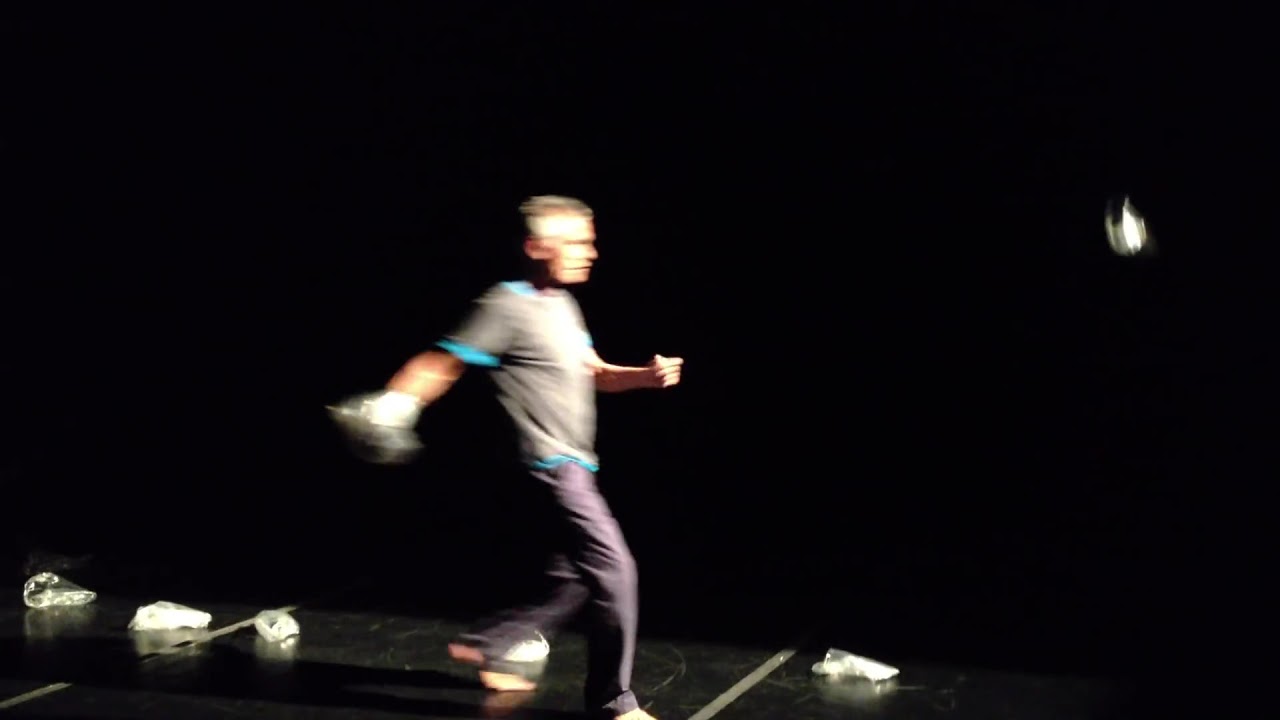The image is a blurry photograph of a man on a black floored stage, illuminated by an off-screen light source from the right, leaving the foreground in pitch darkness. The man, whose short hair is barely discernable, is facing right and appears to be in motion, possibly throwing a clear plastic bag containing a white object with his right hand. His left arm is pointed forward while his right arm is positioned backward. He is wearing purple pants, white tennis shoes, a black t-shirt with blue edging, and a blue undershirt. Near his left foot lies an orange sack. The stage floor features some gray diagonal lines and is cluttered with several clear plastic bags, especially concentrated on the left side. One plastic bag is visibly floating in mid-air at the top right of the image.